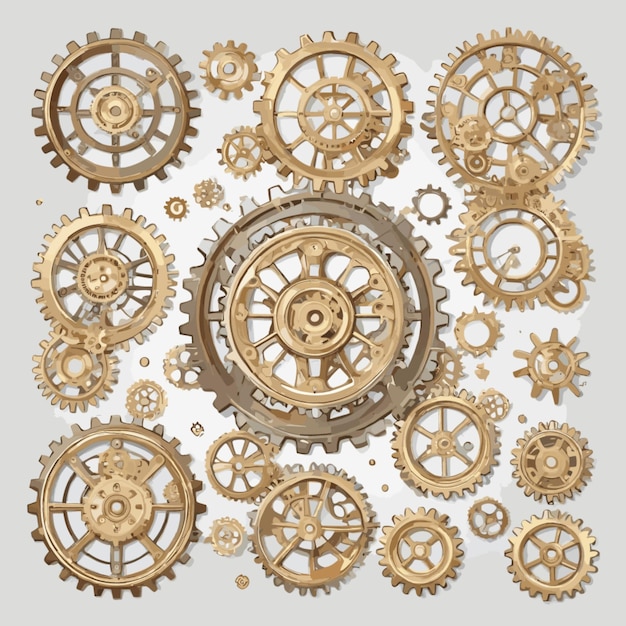This image features a meticulously detailed arrangement of variously sized gears, primarily in shades of gold and bronze. The largest gear occupies the center, distinguished by its golden core and an outer ring shaded in dark brownish-brass. Surrounding it, positioned at the top left, top right, and bottom left corners, are slightly smaller cogs, each contributing to the intricate mechanical tapestry. Scattered throughout the photo are additional gears, all uniformly colored in light gold against a gradient background that transitions from white to very light gray. The gears display a range of designs, including some with spiky spokes and others with nested smaller gears. The overall composition suggests a computer-generated origin, emphasizing the precision and uniformity of the myriad mechanisms presented.